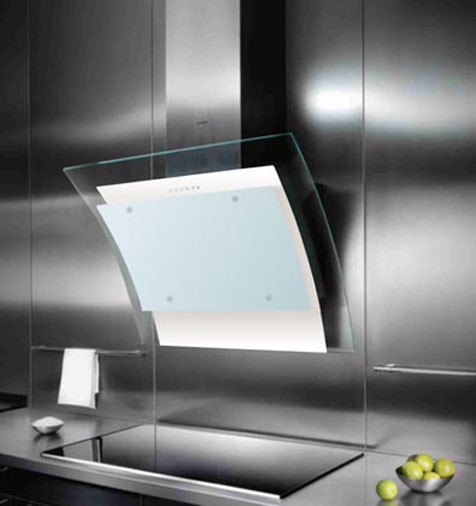This image portrays a futuristic, ultra-modern kitchen setup featuring a sleek, metallic background in shades of black, grey, and silver. Dominating the center is a large, shiny basin without visible faucets, adding to the minimalist design. To its left hangs a small white hand towel, and nearby sits a silver bowl filled with an indeterminate white material, possibly sugar or salt. To the right, a metal bowl holds green limes, adding a pop of color to the otherwise monochrome scene.

In the middle of this setup stands an intriguing, clear glass screen, resembling a futuristic computer or smart touchscreen device. This translucent panel has a light blue section within it, enhancing its high-tech appearance. Directly underneath the screen, a reflection is visible, suggesting the presence of another screen or reflective surface.

The overall composition merges real and surreal elements, presenting a space that is both sophisticated and ambiguous, inviting the viewer to interpret its exact nature.